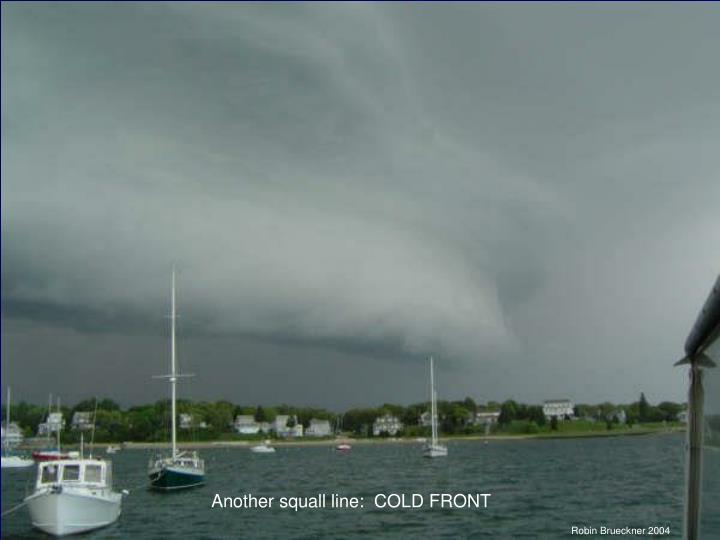The image depicts a group of boats floating on a calm waterway under a dramatic, stormy sky. The sky is an ominous gray, dominated by an enormous, cottony storm cloud that appears to hover close to the water, indicating the approach of severe weather. The boats, varying in design and color, are scattered across the water. In the bottom left corner, a white boat with three windows is prominent. To its right, another boat stands out with a dark green bottom, a white top, and a tall, sail-less mast. Further back and closer to the shore, white and red boats add to the scene's diversity. The shoreline behind the boats is lined with white and gray houses interspersed with lush trees. The sky covers the top two-thirds of the image, emphasizing the looming storm. At the bottom of the picture, white text reads "Another squall line, COLD FRONT," with "COLD FRONT" in uppercase Arial sans-serif font. In the bottom right corner, the text "Robin Bruckner, 2004" is inscribed, attributing the artwork.